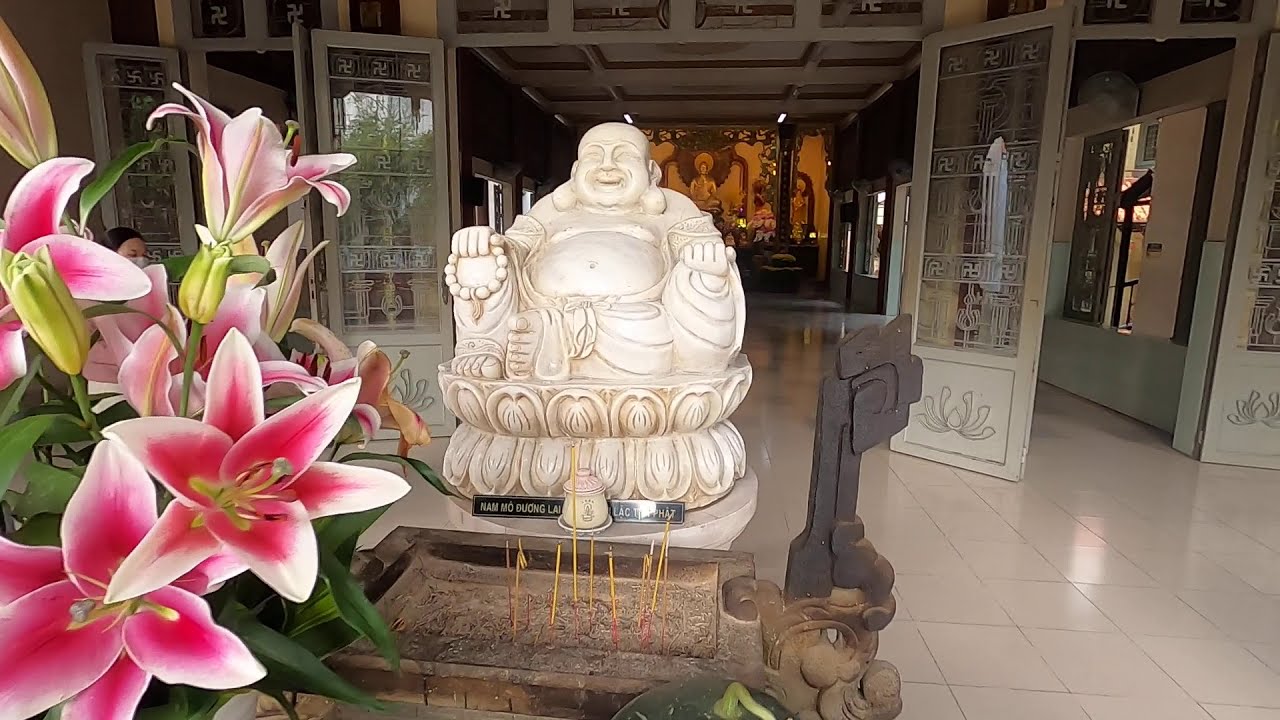The image is a horizontally aligned rectangular photo capturing a serene, large Buddha statue in the center. This white, marble statue depicts a smiling Buddha with a prominent belly and visible belly button. His right hand is holding a beaded necklace or bracelet, while his left hand is palm up, open in a gesture of giving or teaching. The statue, round and gleaming, is perched on a cream and tan marble pedestal. Below the statue, there is a black rectangular sign with white lettering that is not legible in the image.

In the foreground to the left, there are striking pink flowers with white-tipped, pointy petals nestled among green leaves. Behind the Buddha, there are beautiful glass pane doors with intricate patterns and symbols on their light brown or gray frames, suggesting an entrance to a significant place, possibly a shrine or an Asian restaurant.

In the background, another statue can be seen against a brown wall, and there are religious symbols present, possibly Hindu in origin. The floor is paved with square tiles in shades of gray and white. The scene suggests a tranquil and sacred atmosphere, with hints of cultural and religious elements. Additionally, a young Asian woman, possibly wearing a mask, is slightly visible behind the flowers on the left, adding a subtle human presence to the otherwise still and contemplative setting.